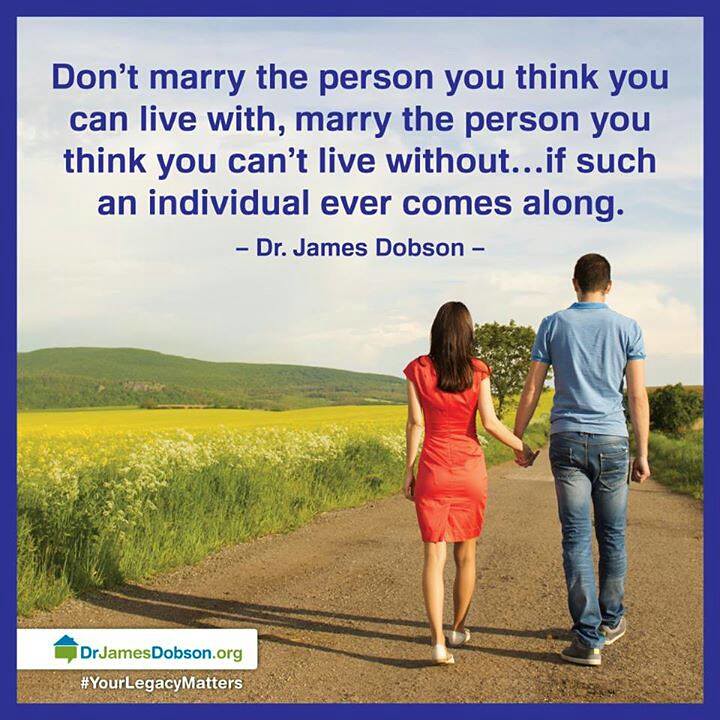The detailed image from drjamesdobson.org titled "Your Legacy Matters" features a memorable quote by Dr. James Dobson in blue text set against a sky background at the top. The text reads: "Don't marry the person you think you can live with. Marry the person you think you can't live without, if such an individual ever comes along." Below the quote is Dr. James Dobson's name. The bottom right quadrant of the image portrays a couple, viewed from the back, walking hand-in-hand down a dirt road. The woman on the left is dressed in a red dress with shoulder-length dark hair, while the man on the right, wearing a blue polo shirt and blue jeans, has short dark hair. Both individuals appear to be walking through a serene natural landscape with green grass, hills, and trees visible. In the bottom left corner, the image displays the logo "drjamesdobson.org” alongside the text "#YourLegacyMatters." The picture is framed with a blue border, adding an additional touch of cohesion to the overall design.